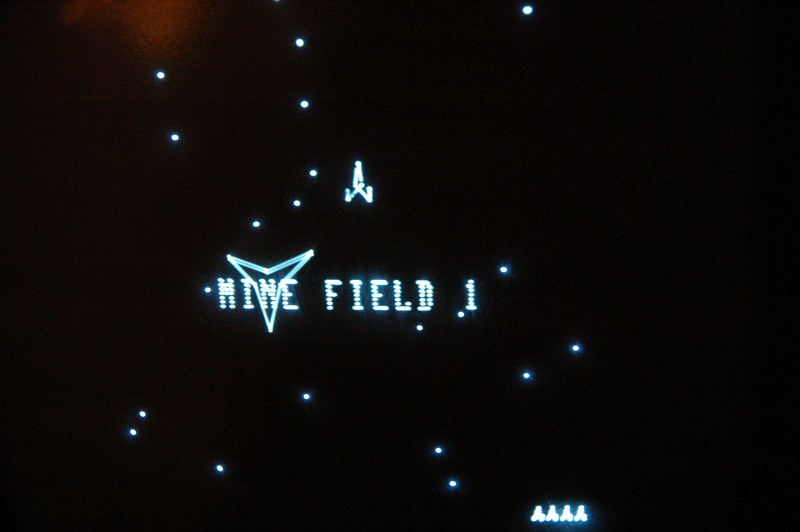This image appears to be a screenshot of an old-fashioned computer game titled "Minefield One." Dominated by a solid black background, the screen displays various elements in light blue, almost a faded blue color. In the center, illuminated letters spell out "MINEFIELD ONE" with a triangular-like logo behind the text. Above these words is a simple, rocket-shaped figure pointing upwards, characterized by a small pointer with a couple of V-shapes beneath it, resembling boosters. Scattered across the screen are numerous neon-colored dots, appearing like stars in space, numbering around 15 in total. In the bottom right corner, there are four small triangle figures, representing the player's lives. The overall aesthetic suggests a vintage game from the late 70s or early 80s, reminiscent of classic space shooter games, with a minimalist, retro design palette of blue and white against a predominantly black backdrop, and a subtle orange haze in the upper left corner.